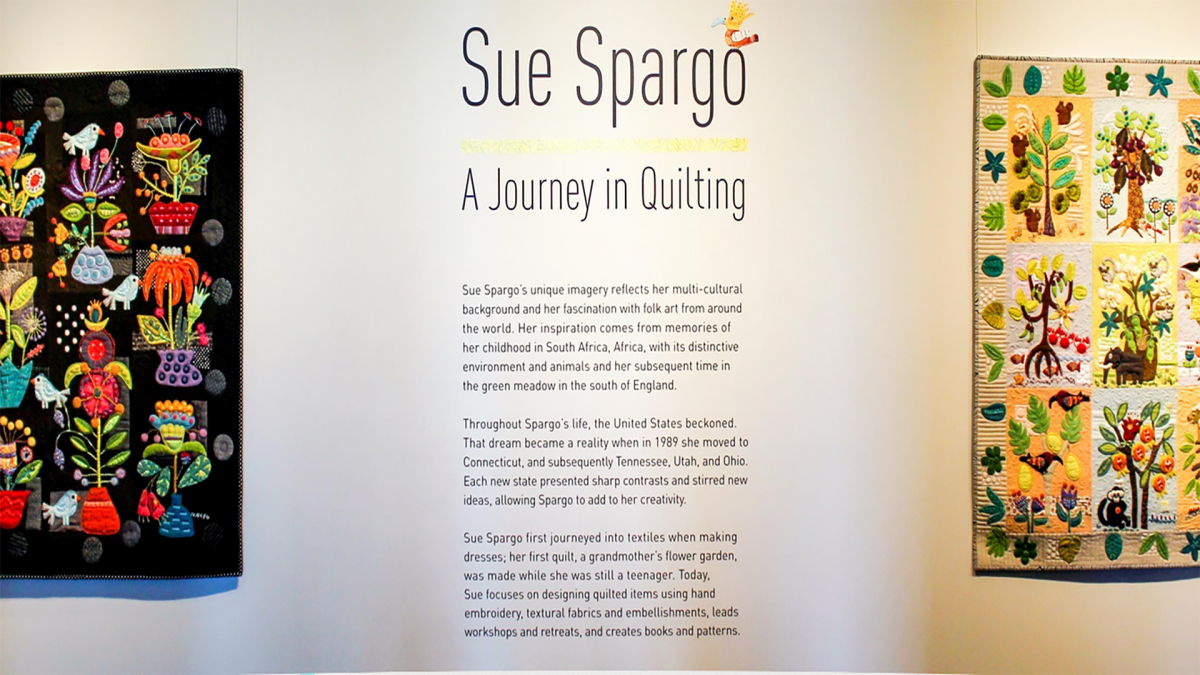The poster depicts a display likely found in a museum or gallery, showcasing two quilts by Sue Spargo, accompanied by detailed textual information about the artist and her work. Dominating the poster is the title "Sue Spargo, A Journey in Quilting," followed by several paragraphs elaborating on how her unique imagery is influenced by her multicultural background and fascination with global folk art. The display includes two quilts: on the left side, a vibrant quilt set against a red and purple background, featuring numerous small, colorful images like pots of flowers and arrows. The right-side quilt predominantly features yellowish-white tones with brown and green flowers. The poster itself has a gray background, creating a cohesive frame for these intricate and varied artworks that reflect Sue Spargo's artistic journey.